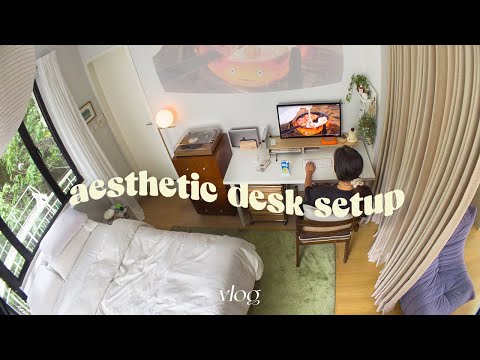An aerial photograph of a bedroom showcases a person with black hair wearing a brown t-shirt, seated at a white desk with a wooden chair. In front of them is a large computer monitor displaying an image, which is also projected on the wall. To the left of the desk is a black dresser with a record player on top. The room features a bed with white sheets and pillows under a window with black trim and white curtains, revealing lush greenery outside. There's a green soft rug partially under the bed and a doorway on the adjacent wall. The scene includes a variety of objects such as a white keyboard, a plant, a lamp, and a large portrait print on the wall. The image has a GoPro feel and is bordered by solid black strips at the top and bottom, giving it a distinctive, framed look. The caption on the wall reads "Aesthetic Desk Setup."